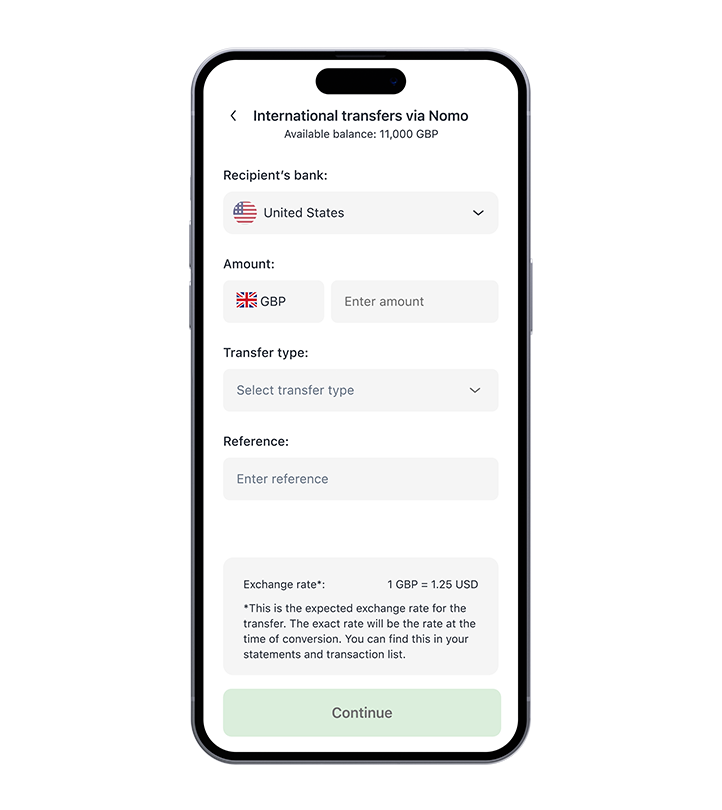Screenshot of a NOMO International Transfer Interface

The screenshot shows an interface for initiating an international money transfer via NOMO. The available balance displayed is £11,000 GBP. The recipient's bank country is selected as the United States from a drop-down menu. The transfer amount is specified in GBP, with an entry field available next to the selection.

Below the amount entry section, there is an option to select a transfer type via another drop-down menu (specific options are not visible in the screenshot). 

Further down, there is a field labeled "Reference" where users can enter a reference number to identify the transaction. This reference is crucial for tracking and ensuring the correct recipient picks up or receives the funds.

The exchange rate provided is 1 GBP = 1.25 USD, indicating the expected rate at the time of this transfer. This rate is subject to change until the exact moment of conversion, with the final rate available in the user's statements and transaction list.

At the bottom of the interface, there is a green "Continue" button to proceed with the transfer process.